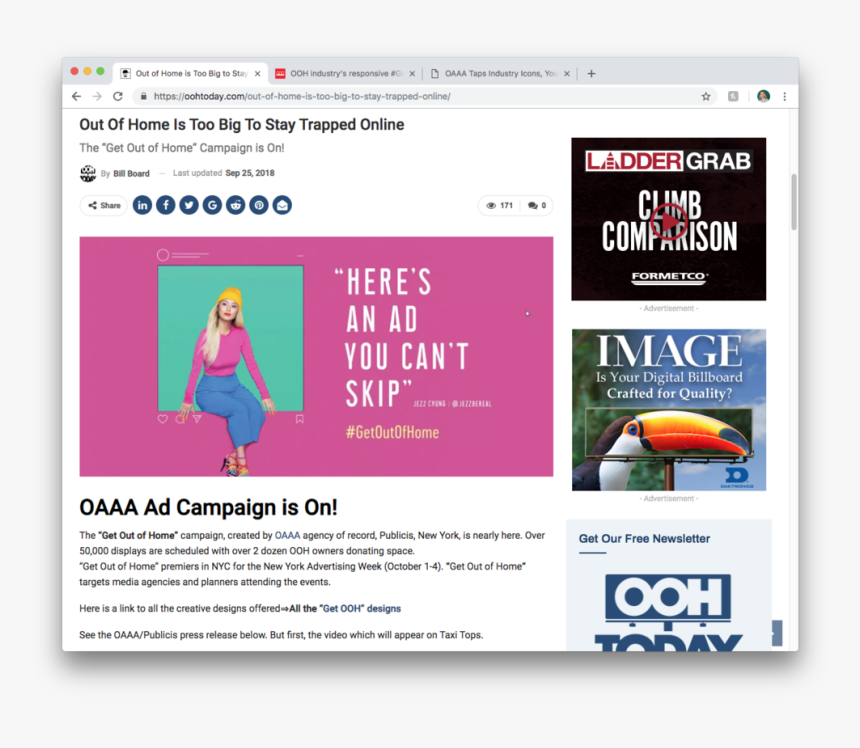Screenshot of a computer monitor displaying the website eToday.com. At the top, a gray bar hosts three dots on the left—red, yellow, and green—with the red one indicating the active tab. The active tab reads "Atomhome is too big to ST," while the two background tabs are titled "OO Industry Responsive" and "OAAA tapped industry icons."

Below the tabs, the URL bar features navigation buttons including a reload icon and a back arrow to the left. The main webpage is predominantly white, with bold black text stating, "Atomhome is too big to stay trapped online. The Get Out of Home campaign is on," authored by Bill Board. A note on the right reads, "Why Not Update?" with the date, September 25, 2018.

Underneath, a row of dark blue social media icons offers sharing options via Share, Instagram, Indeed, Facebook, Twitter, Google, Reddit, and Email. To the right of these icons, an open eye icon displays the number 171.

The center of the page features a pink box with white text stating, "Here's an email from Get Out of Home" alongside a yellow hashtag. Adjacent, a cyan-colored square displays an illustration of a girl with yellow hair, wearing blue bottoms, seated at the bottom of the square. Next to this image, text reads "OAAA Ad Campaign," followed by a descriptive paragraph.

On the right side of the page, three advertisements are visible. At the very bottom of the image, a dark blue text on a gray background prompts users to "Get our free newsletter" from eToday.